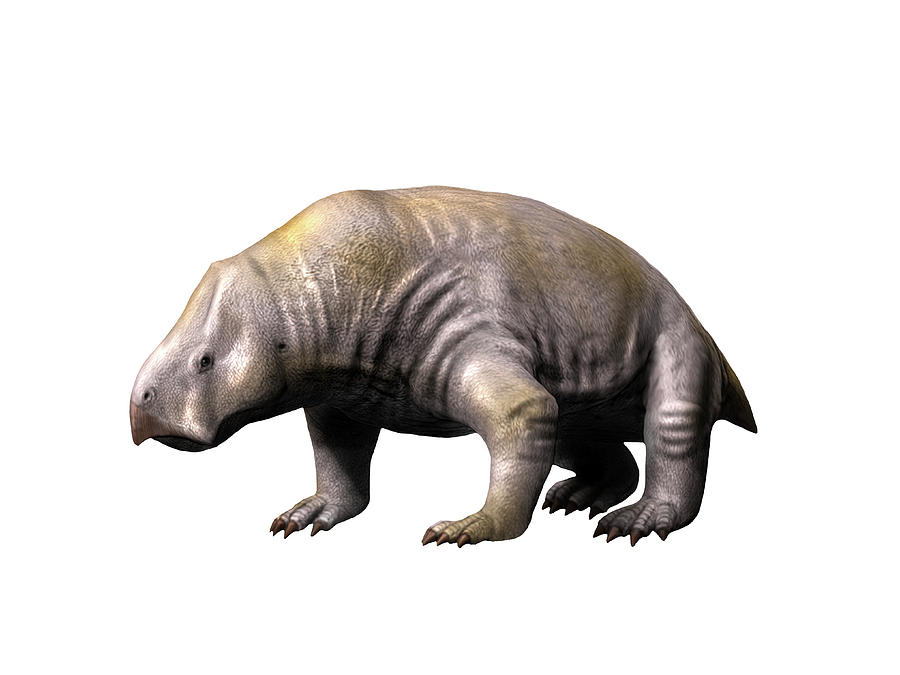This highly detailed CGI image depicts a fantastical creature with distinctive characteristics. The creature boasts gray skin with hints of light brown coloration, and a large, robust, and muscular body that hints at immense strength. Its head features a short, pointy beak, small beady black eyes, a tiny nose hole, and a small ear hole, giving it a hybrid appearance reminiscent of various animals. It stands hunched over with its elbows jutting outward, and its powerful, clawed feet augment its formidable look. The creature has a thick, round physique similar to that of a walrus or a rhinoceros without a horn, complemented by a short, pointed tail. The background of the image is stark white, further highlighting the creature's unique and imaginative form, which combines elements of prehistoric and otherworldly designs.